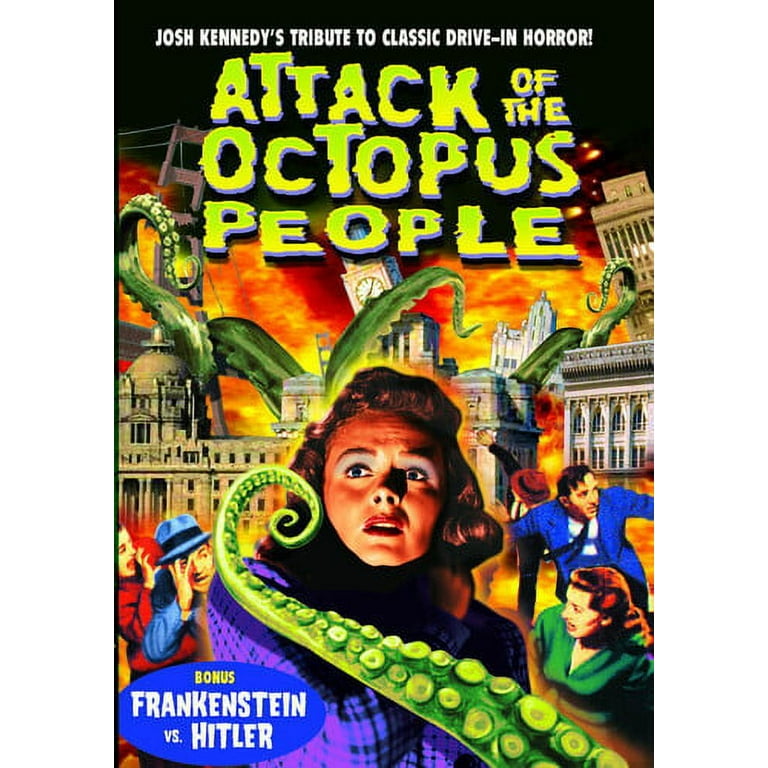The book cover, designed in a cartoon realist style, vividly portrays chaos and horror. The top third of the cover is black with white text that reads "Josh Candy's Tribute to Classic Drive-In Horror." Below it, in a distressed neon green horror font, the title "Attack of the Octopus People" stands out. The scene below is one of terror: the Golden Gate Bridge is being torn in half, Big Ben is collapsing, and other buildings are crumbling amidst a backdrop of towering flames. Bright green octopus tentacles, complete with detailed suckers, emerge from the destruction, wreaking havoc.

In the foreground, a woman with a terrified expression is prominently featured, with a green tentacle menacingly poised near her. Surrounding her are five other frantic individuals – three on the right and two on the left. The people, dressed in 1960s-style attire, are depicted running and screaming in fear. The man on the left wears a blue suit, and the woman beside him is in a green dress. The bottom-left corner of the cover features a blue oval with the word "Bonus" in yellow print, and beneath it, "Frankenstein vs. Hitler" in white, highlighting an added feature.